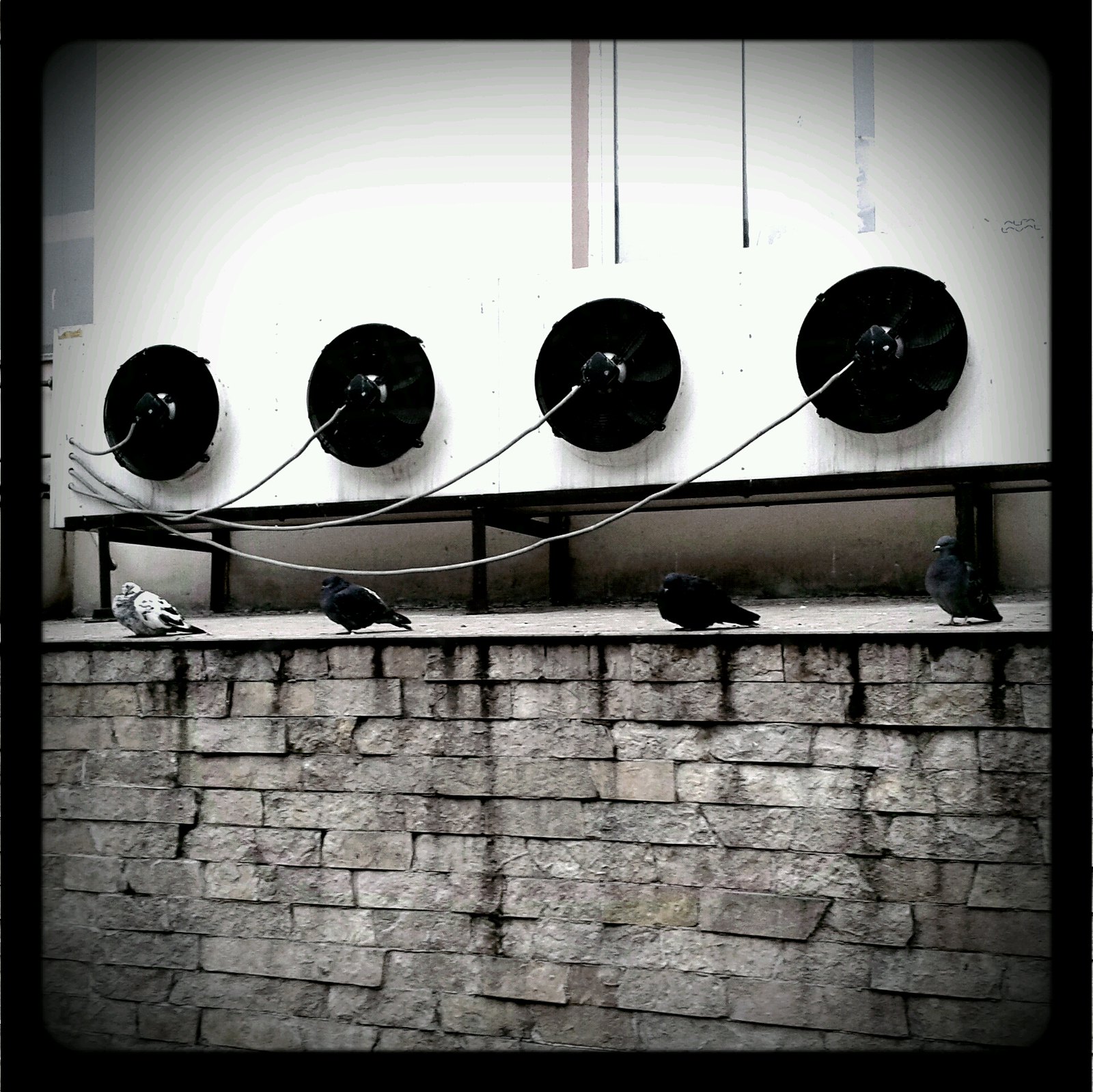The image is a black and white photograph framed by a thin black border. The scene depicts a gray stone wall, constructed from tightly arranged bricks that resemble stone. Atop this wall, there is a white ledge where four pigeons are perched. The first pigeon on the left is speckled white and black, while the remaining three are predominantly black with tiny white tips on their beaks. Above the birds, there's a white rectangular structure featuring four black circular disks, each with wires extending from their centers and disappearing off the left edge of the frame. The uppermost part showcases another section of the building, a white wall adorned with vertical stripes. The overall composition exudes a sense of symmetry and harmony, accentuated by the orderly arrangement of the birds and circular disks.